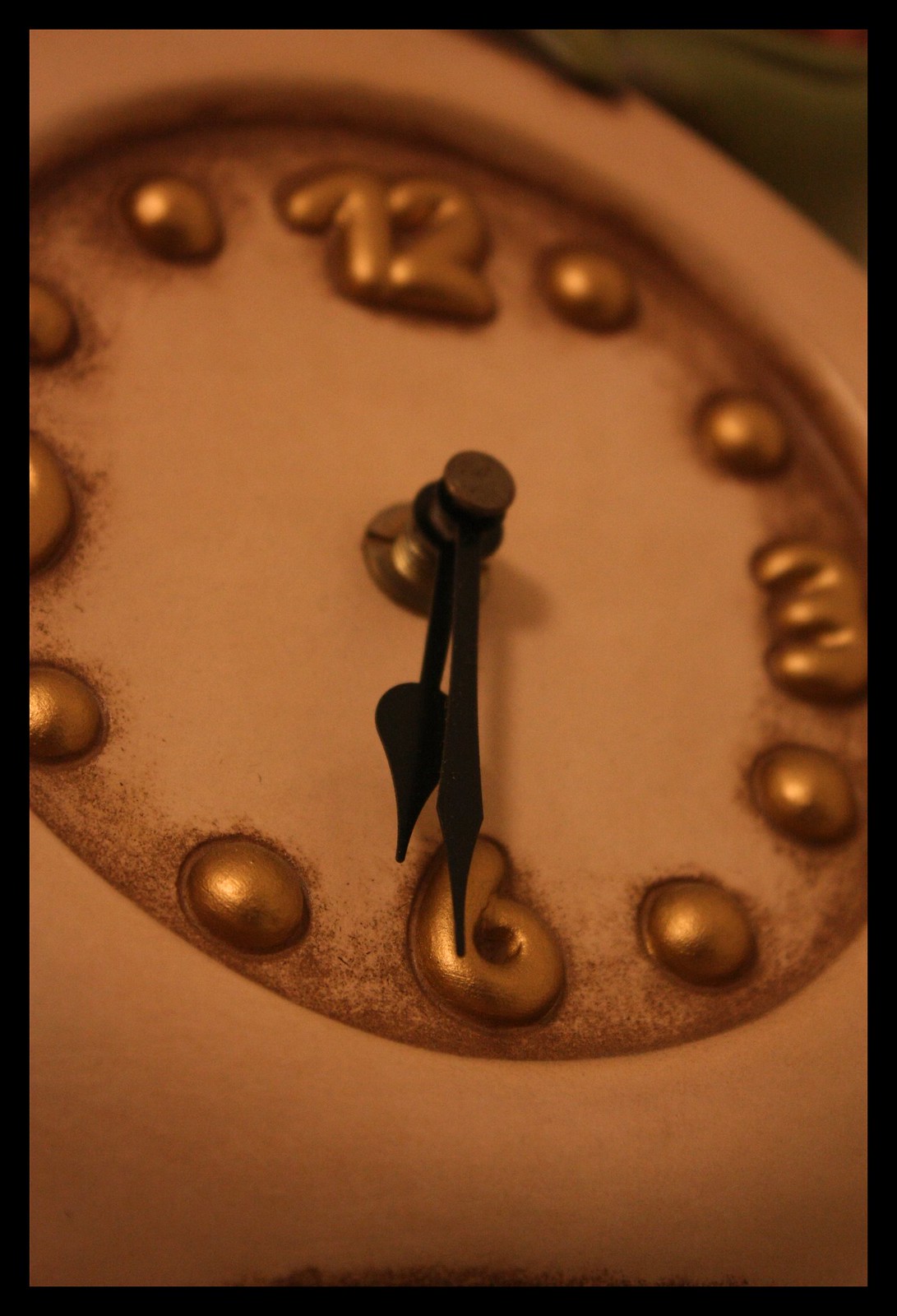Close-up of an antique-style round clock with an elegant design. The image features a filter that gives the clock a rusty brown tint, enhancing its vintage aesthetic. The clock's outer casing is white, as is its face, which is accentuated with black hands. Only the numbers 12, 3, 6, and 9 are prominently displayed, each in a bold, gold-colored, thick-font style. The remaining hours are marked by small, gold-colored round balls. A subtle touch of brown dust appears brushed around the numbers on the clock's white background, contributing to its aged and nostalgic appearance.